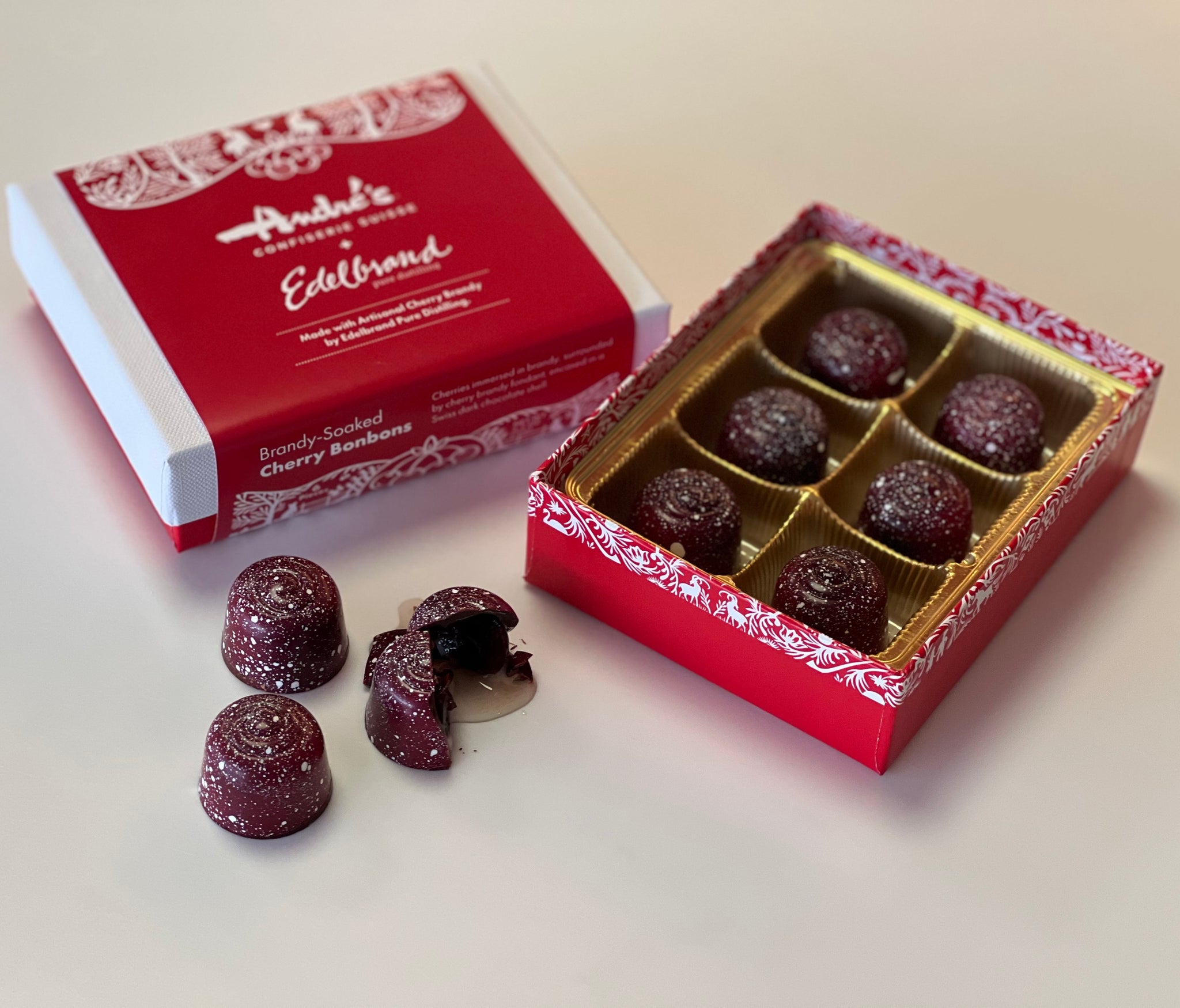This image features a beautifully arranged box of chocolates displayed on a white background, with soft shadows cast from the top left corner to the bottom right. Central to the composition is an elegant box of cherry bonbons, branded “Andres Edelbrand,” which prominently displays the text “brandy-soaked cherry bonbons.” The box, adorned with a festive red and white cover that may feature a Christmas-like design with reindeer, holds six dark red chocolates within a gold plastic tray, each candy nestled in its own compartment.

To the side, three of these circular chocolates rest on the white surface. Among them, two remain whole while the third is split open, revealing a glossy, semi-clear liquid seeping out, likely from the brandy-soaked cherry inside. The chocolates have a dark red coating sprinkled with tiny white speckles, adding to their sophisticated appearance. The meticulously crafted presentation and vivid colors of this image evoke a sense of luxury and indulgence.